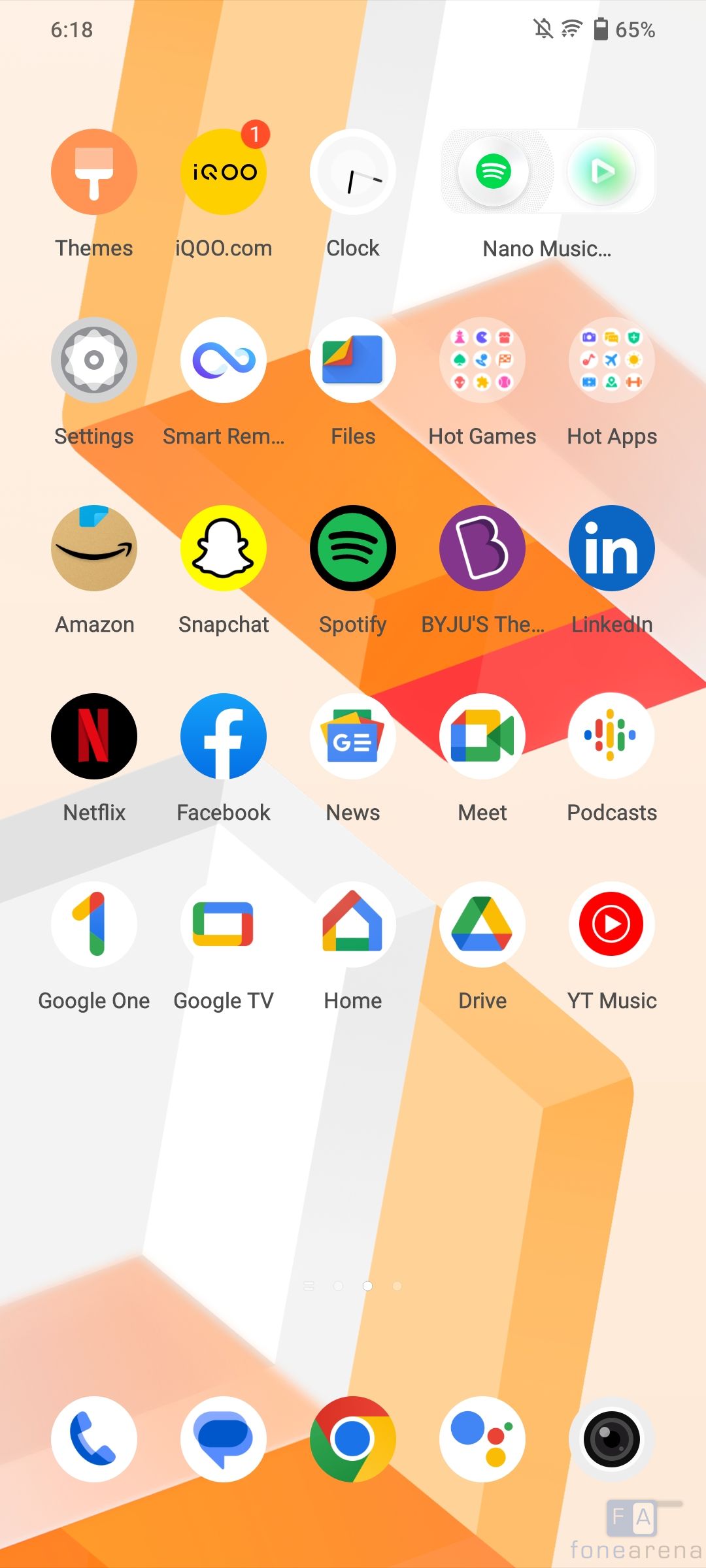This image is a detailed screenshot of a smartphone home screen. The background features an abstract artwork comprised of diagonal rectangles in varying shades of orange, white, and gray. At the top right corner of the screen, the time is displayed as 6:18, accompanied by a notification bell with a slash through it, an icon signifying wireless connectivity, and a vertical battery icon showing 65%.

The screen is organized into a grid with five rows of five circular app icons, filling up approximately the top two-thirds of the display. Below this, a dock of five more circular icons spans horizontally across the bottom. Each app icon is labeled in a dark font underneath, with names such as Themes, iqoo.com, Amazon, Snapchat, Spotify, Meet, Podcasts, Google TV, Netflix, and Facebook visible among others. Some icons, such as Hot Games and Hot Apps, contain smaller sub-icons in multiple colors like green, blue, red, orange, and yellow.

The app icons are visually distinctive: Spotify features a green circle with black sound waves, Amazon showcases a brown box with a black smile and a hint of blue, and Facebook is represented by its iconic round blue circle with a white 'F'. The bottom dock includes, from left to right, a telephone icon, a chat icon, the Google Chrome icon, a Google app icon with multicolored dots, and a final icon resembling a black eyeball.

At the very bottom right corner of the screenshot, there is a faint watermark that reads "Phone Arena," with a shaded logo featuring the letters 'F' and 'A' positioned directly above the text.